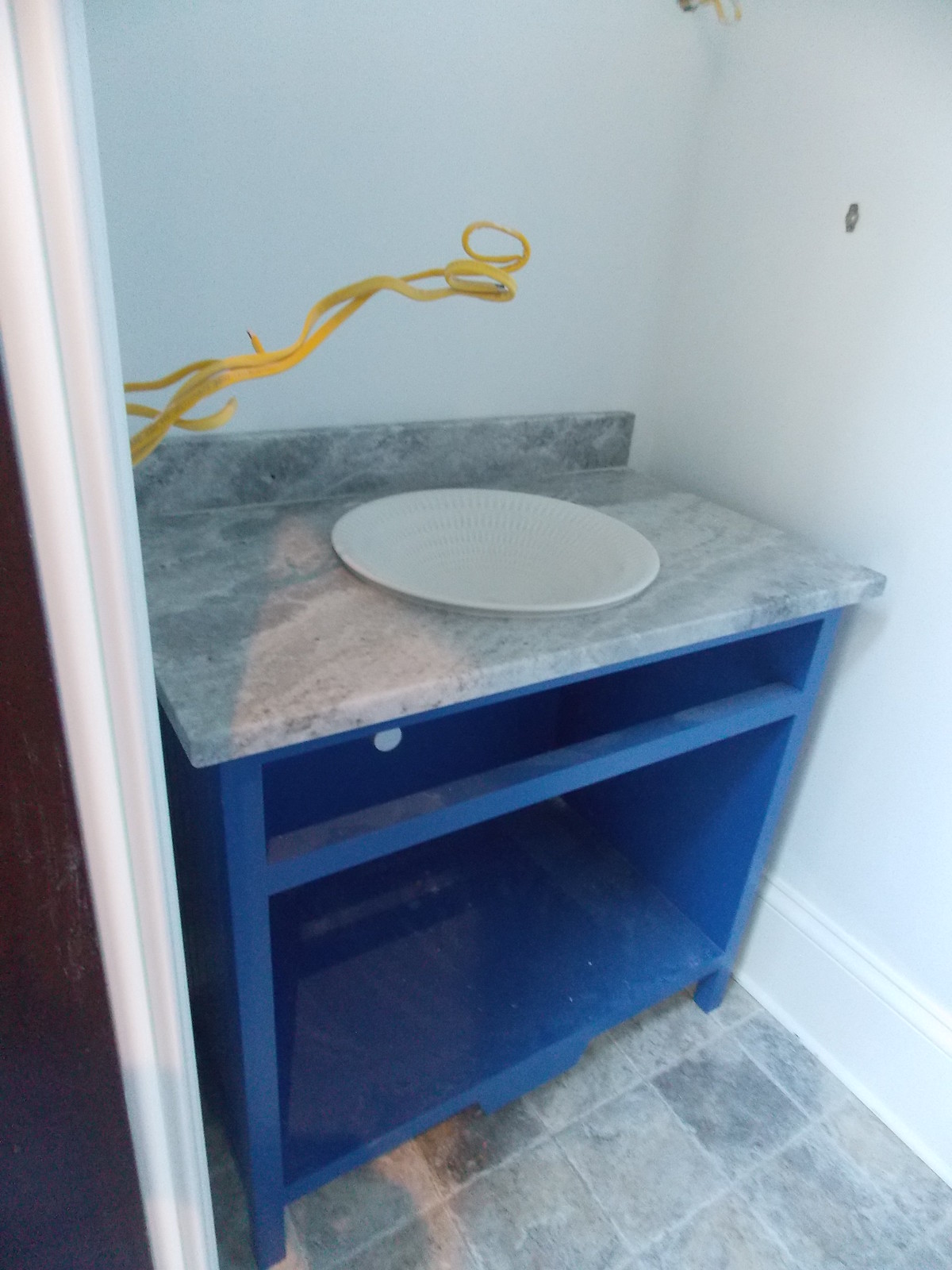A bathroom under construction features a marble tabletop with intricate gray-white designs, set against a white wall. Emerging from the left side of the wall, a yellow wire, possibly an ethernet cable, lies unattached. Below the tabletop is blue shelving, which provides a stark contrast to the white walls and brings a pop of color to the unfinished space. A white post with a wooden front stands on the left side, supporting part of the structure. The floor is tiled, marking the base of this work-in-progress bathroom. Notably, there are no pipes or sink installed yet, and a clip is attached to the right wall, hinting at ongoing construction work.